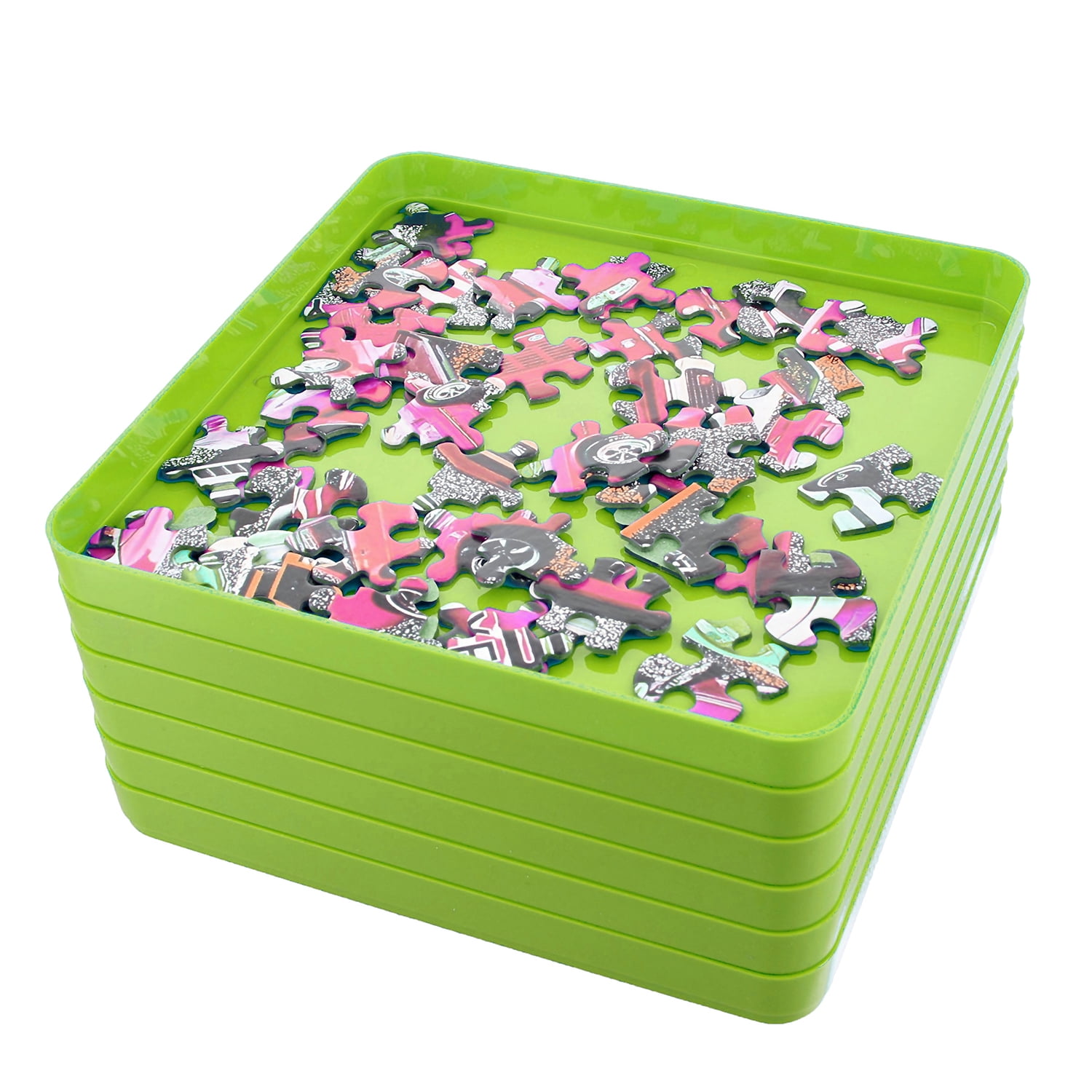This color photograph showcases six lime green, plastic trays stacked atop one another against a plain white background. Each tray is shallow, about an inch deep, and designed for organizing jigsaw puzzle pieces. The trays are positioned slightly at an angle, providing a side view that highlights their layered arrangement. The topmost tray contains an assortment of puzzle pieces predominantly colored in shades of pink, black, white, light blue, gray, and purple. The image, likely meant for stock photography, captures the organized nature of the trays, suggesting an efficient way to manage puzzle pieces based on their colors. There is no text visible anywhere in the image.